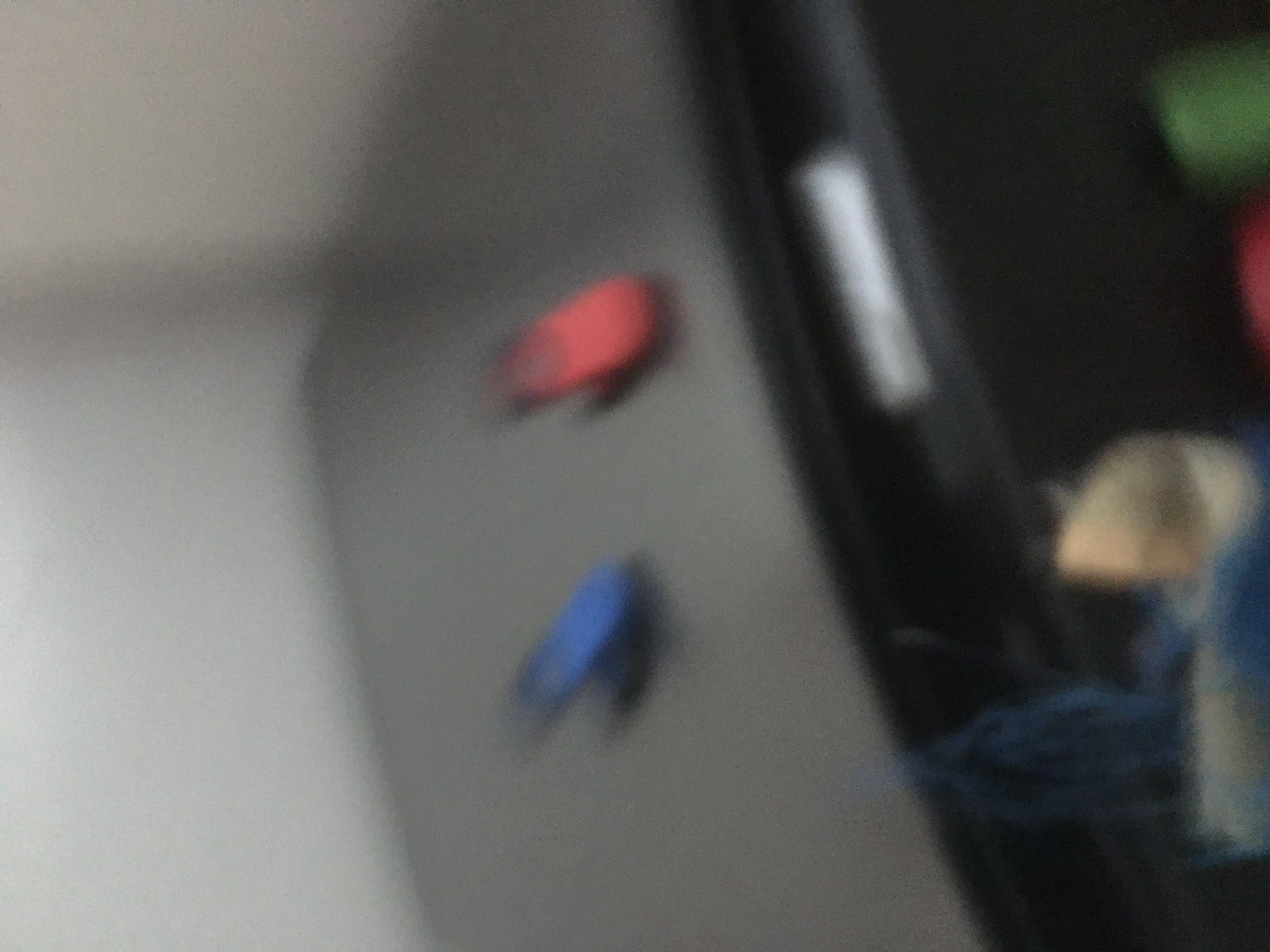In this extremely blurry and out-of-focus photo, discernible features appear as geometric shapes and color blocks. On the left side, there's a light gray area resembling part of a wall with a baseboard and white floor tiles. Adjacent to this on the right is a dark gray object with a red button on top and a blue one below it, next to a black strip. The object also has a white rectangular sticker or tag on its side. In the lower right corner sits a golden object encircled by a bluish halo, with strands of blue appearing to blow out to the side. Above, there are distinct green and red shapes side by side.